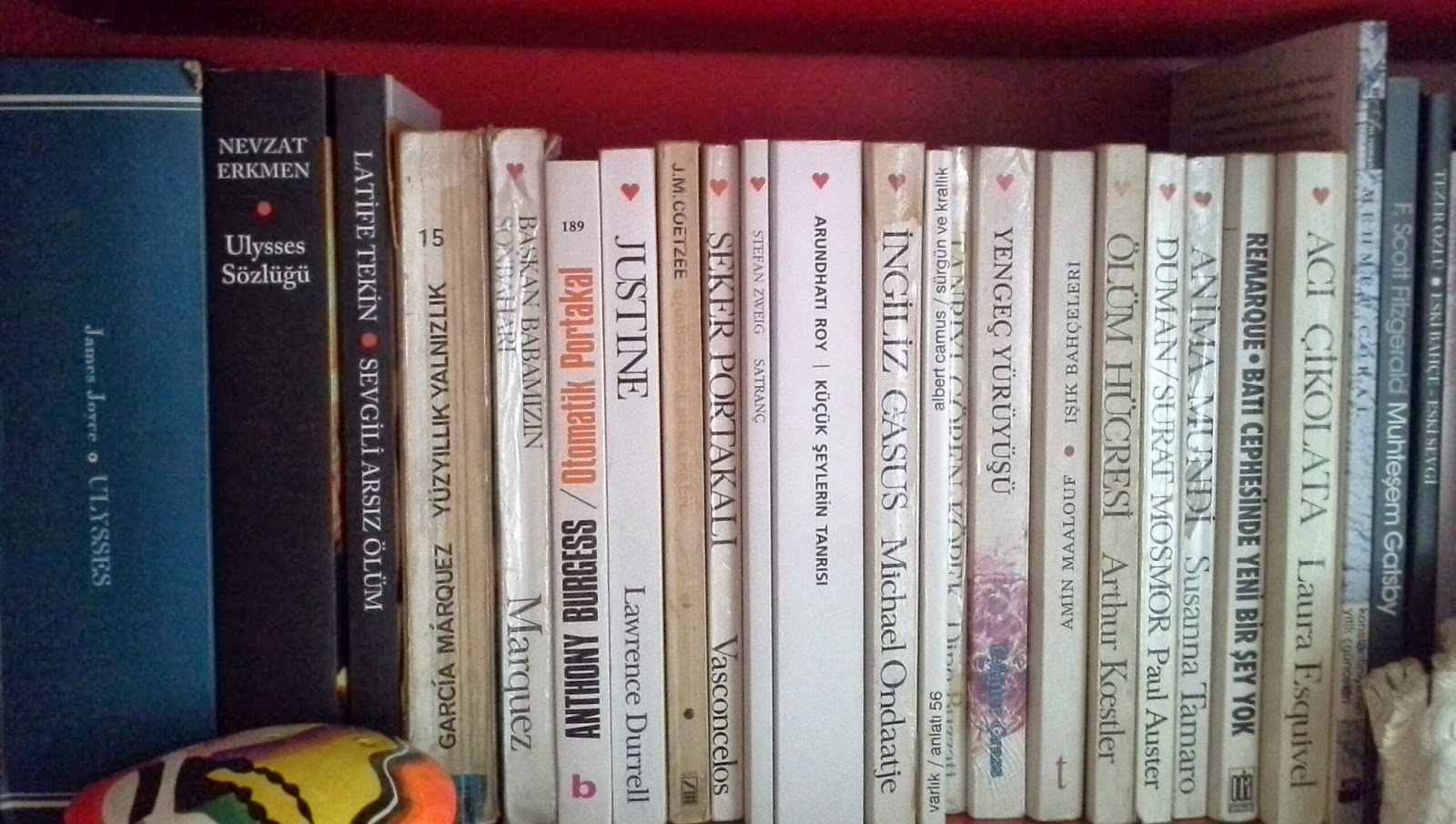The image displays a bookshelf filled with a diverse collection of approximately 24 books, predominantly in a language other than English. The focal point includes notable titles such as "Ulysses" by James Joyce, with another volume or study related to "Ulysses" nearby, and works by Gabriel Garcia Marquez. The books vary in color and thickness, with bindings in shades of blue, black, white, and gray. Positioned in front of the books are a few artifacts, including a small puppet or stuffed animal at the bottom right and a jar on the bottom left. The objects and books are horizontally centered within the frame, suggesting a scene from a home or public library. The background behind the books is faintly red, adding a touch of warmth to the setting.